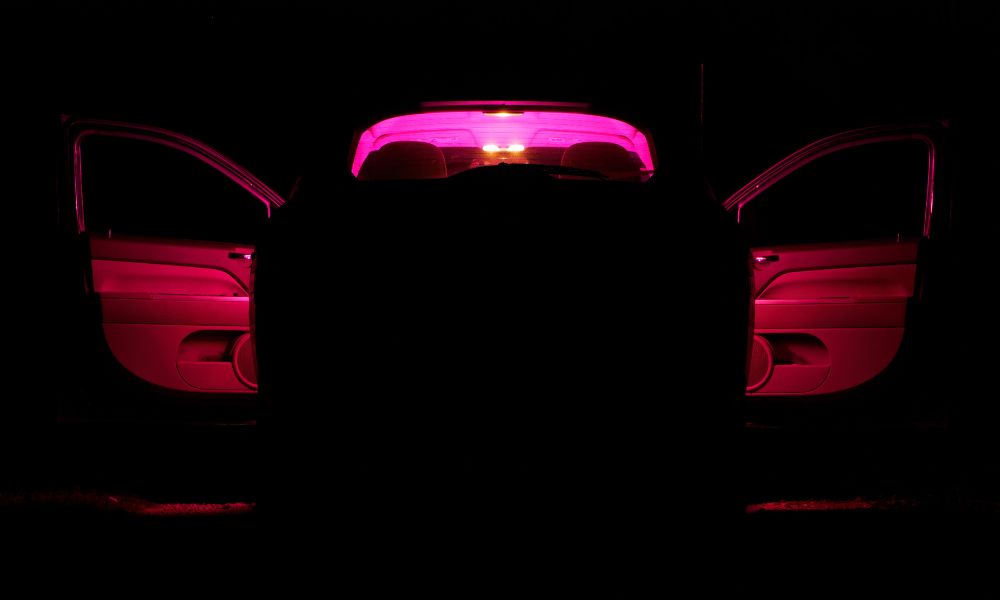The image depicts a dark background with a car as the main subject, illuminated by a distinct purplish hue. Both doors of the vehicle are open, resembling wings, with visible armrests and pockets underneath. The interior is dimly lit, revealing the top backs of the front seats. A light situated on the roof between the seats, emitting a purplish glow, illuminates parts of the interior. The purple light extends to the windshield area, casting a glare off the rear-view mirror. Additional purple hues are seen on the open doors and extend horizontally towards the bottom edges of the image. In the backdrop, there are faint red and pinkish shades mingling with the purplish tones. There's also a silhouette of an indiscernible object, further adding to the mysterious ambiance.